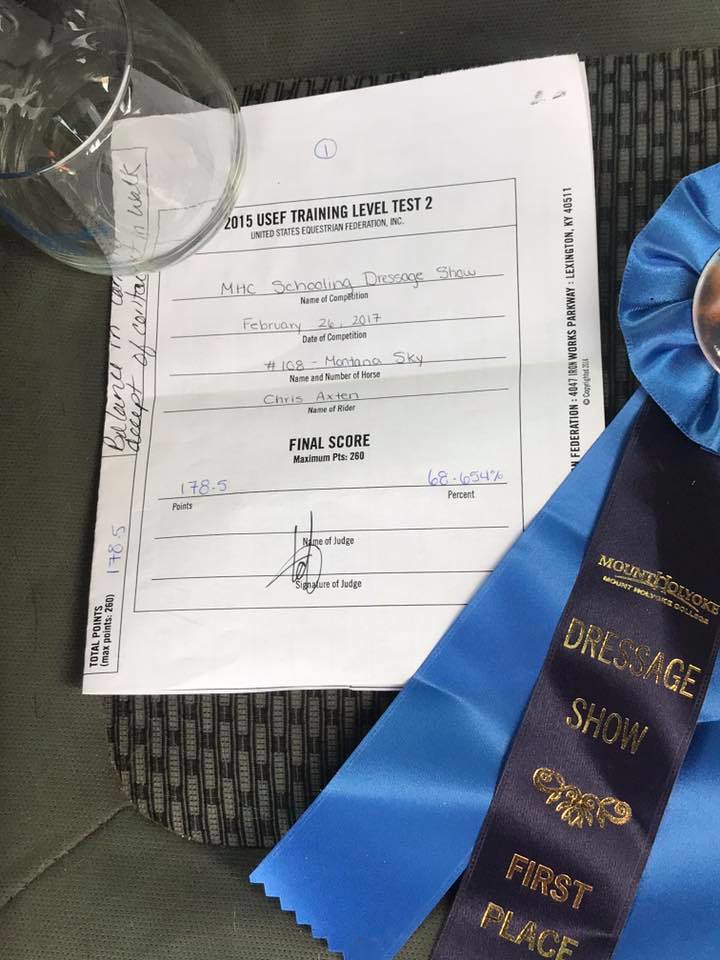In this rectangular photograph, the focus includes several items meticulously placed. Centered on a surface is a white piece of paper with both printed and handwritten details, primarily about a dressage competition. The header on the paper reads "2015 USEF Training Level Test 2," indicating it's an official document from the United States Equestrian Federation. Detailed information includes “MMC Schooling Dressage Show, February 24th, 2017,” the rider's name "Chris Axton," the horse "Montana Sky" with number "108," and a final score of 178.5 points, equating to 68.654%. 

Perched on the top left of the paper is a clear, empty drinking glass. On the right, prominently displayed, is a striking blue ribbon adorned with lighter blue edges and gold lettering. This ribbon announces "Mount Holyoke College Dressage Show - First Place," signifying a celebratory moment of victory. The composition portrays a celebratory sentiment, where the test scores, detailed documentation, and the first-place ribbon collectively underscore an achievement in dressage.